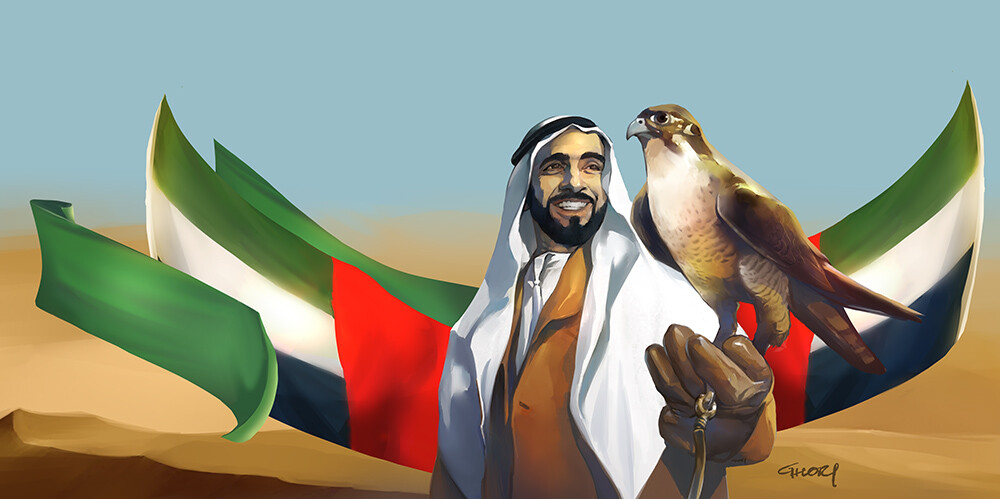The digital artwork depicts an Arab man, identifiable by his traditional white shemagh headdress secured with a black agal (cord), and a tan robe. The man sports a black mustache and beard, and he warmly smiles at a bird perched on his gloved left hand. The bird is predominantly brown with white and green markings and has a short gray beak. The background features flags resembling those of the United Arab Emirates, comprised of horizontal stripes in green, white, and black with a red section along the hoist side, giving the appearance of wings. The top portion of the backdrop is a clear blue sky, while the lower section depicts sandy desert terrain. A signature, somewhat ambiguous and challenging to decipher, appears in the lower right corner, possibly reading "G. Horry."